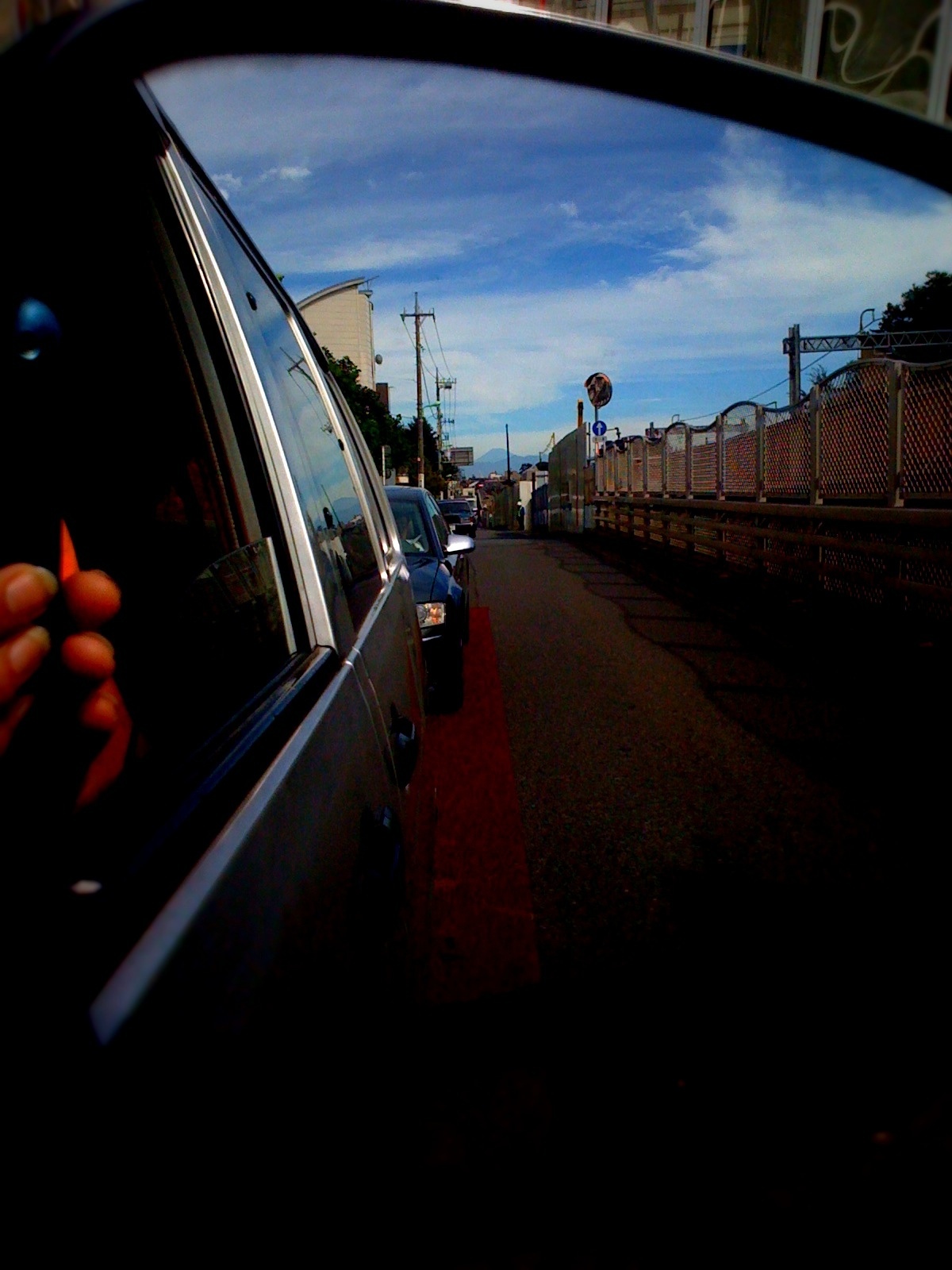This photograph, captured during the daytime from the driver's side of a black sedan, offers a detailed view of a one-way street with a line of black cars following behind. The focal point includes the driver's left hand holding a cell phone out of the open window. The sky above is light blue with large, white clouds scattered across it. Along the right side of the image, a metallic fence with circular wire patterns runs horizontally, separating the street from another area. The scene includes several electrical posts and wires receding into the distance. On the left side, a light-colored, unique-shaped building is visible. The street, although lined with multiple vehicles, doesn't appear overly crowded or busy.